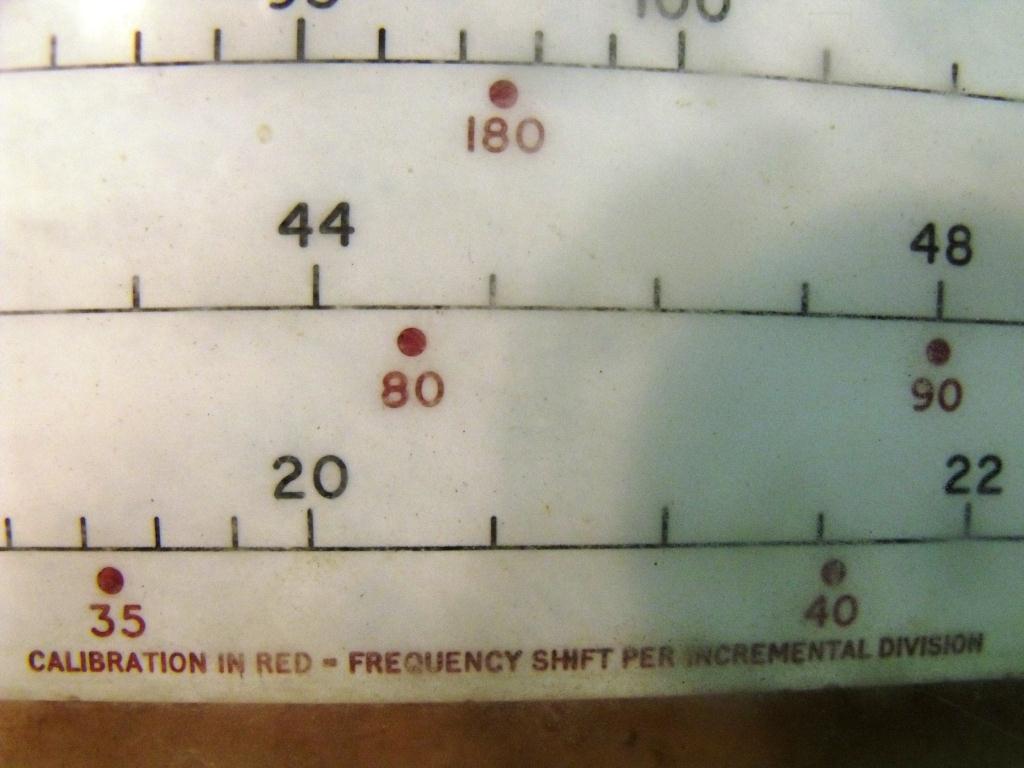This photograph captures a close-up view of an aged, backlit frequency indicator with a tuning dial, reminiscent of a vintage instrument or radio. The title "Calibration" is prominently displayed in red at the top of the screen. The dial features multiple bands, each marked with various numbers and calibrations that exemplify classic design aesthetic.

The screen, made from thick, translucent material, exudes an old-school charm, typical of early electronic devices. The numbers on the dial, distinctly burned onto the surface, highlight their vintage style. Three horizontal graphs with incremental divisions dominate the display. Each graph showcases black numerical indicators, such as 20, 22, 44, 48, 90, and 100, providing reference points for frequency shifts.

In addition to black numbers, there are red calibration numbers - 35, 40, 80, and 180 - that stand out against the translucent background, aiding in precise adjustments. The juxtaposition of red and black numbers against the backlit screen enhances the intricate details, making it a fascinating example of early frequency measurement technology.

Overall, this image is a detailed study of a beautifully aged frequency shift indicator, celebrating the meticulous craftsmanship of bygone eras.